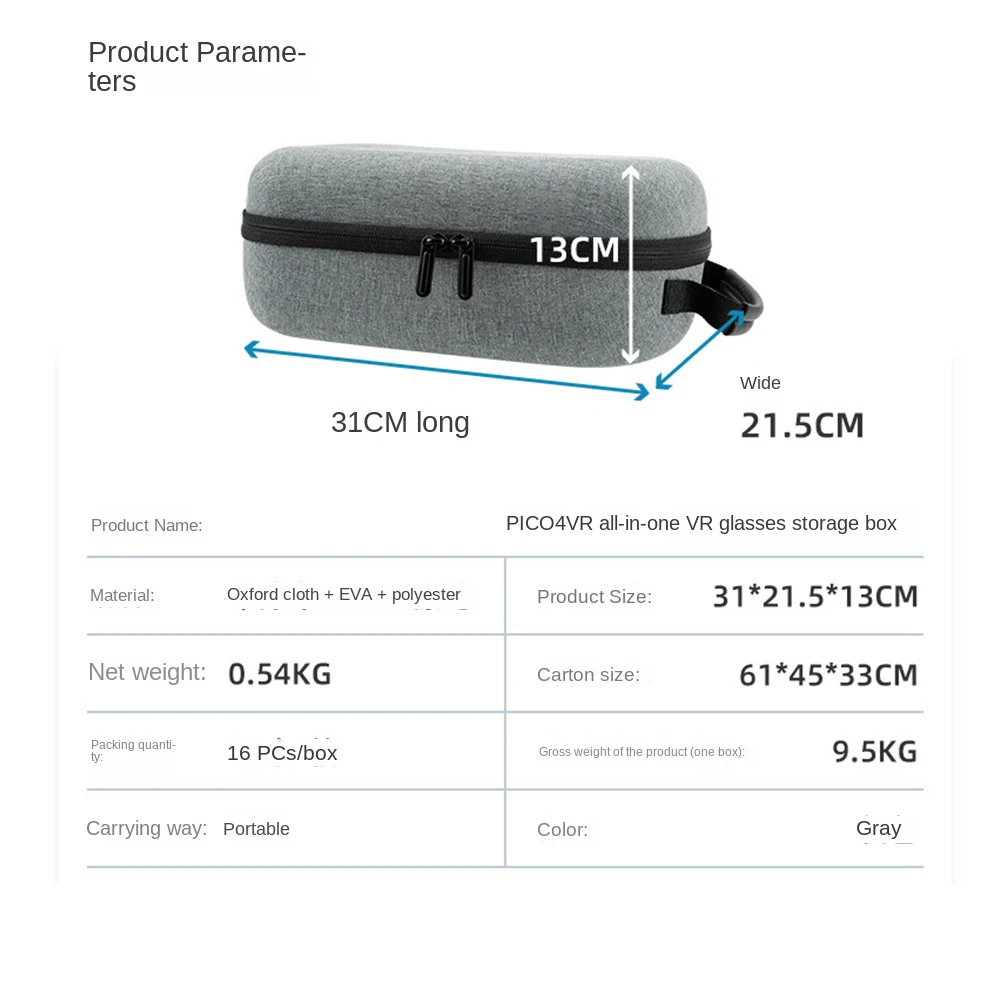The image is a screenshot depicting a detailed specification sheet for a travel case designed to store VR glasses. The title at the top of the image reads "Product Parameters." It provides comprehensive dimensions of the case: 31 cm in length, 21.5 cm in width, and 13 cm in height. The product name is "PICO 4 VR All-in-One VR Glasses Storage Box," indicating its specific use for VR equipment. The material composition of the case includes Oxford cloth, EVA, and polyester. The net weight of the case is 0.54 kilograms. Each box contains 16 pieces of the storage box. The image also mentions that the carrying weight is portable, offering ease of transportation. The product size is reiterated as 31 x 21.5 x 13 centimeters. The carton dimensions are provided as well, measuring 61 x 45 x 33 centimeters, with a gross weight of 9.5 kilograms. The color of the storage box is specified as green. The entire image is presented in a square format with a white background.